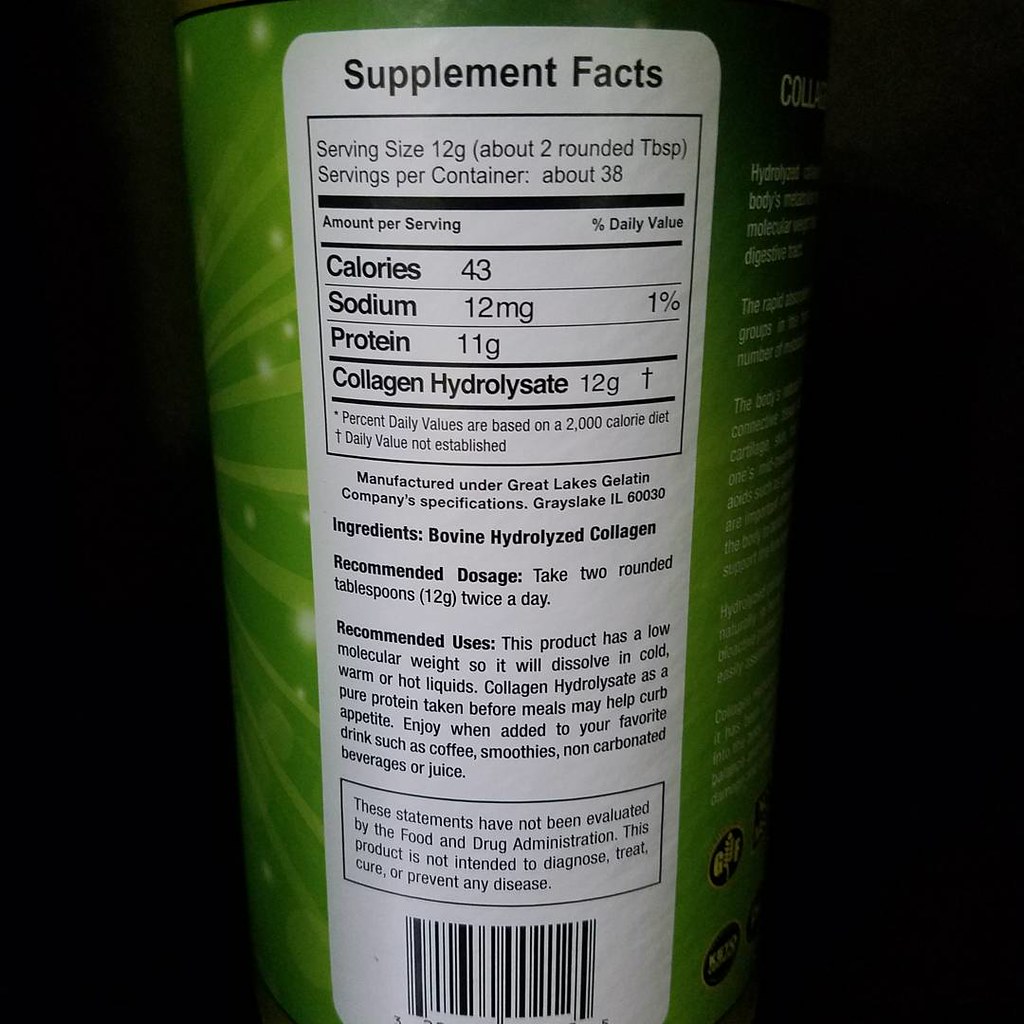The image is a closeup, vertical photograph of a green bottle from the Great Lakes Gelatin Company, displaying detailed supplement information. The bottle prominently features a white nutrition panel with black text that reads "Supplement Facts." The serving size is 12 grams, approximately two rounded tablespoons, with about 38 servings per container. Each serving provides 43 calories, 12 milligrams of sodium (1% of the daily value), and 11 grams of protein, specifically collagen hydrolysate. The bottle also specifies the product is manufactured in Grays Lake, Illinois, under Great Lakes Gelatin Company specifications. The ingredients list mentions bovine hydrolyzed collagen, and the recommended dosage is two rounded tablespoons (12 grams) taken twice daily. The product can dissolve in cold, warm, or hot liquids and may help curb appetite when consumed as a pure protein before meals. Suggested uses include adding it to coffee, smoothies, non-carbonated beverages, or juice. A disclaimer notes that these statements have not been evaluated by the Food and Drug Administration, and the product is not intended to diagnose, treat, cure, or prevent any disease. The bottom edge of the image shows a barcode, partially cut off.